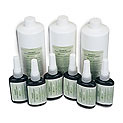In this small image, the focus is on a total of nine bottles arranged against a completely white background. The back row features three larger cylindrical white plastic bottles, each adorned with a yellowish-green label bearing black writing. These bottles tower over the six smaller bottles in the foreground. The smaller bottles, reminiscent of droppers or squeeze bottles with spout tops and white caps, are translucent with a dark black hue. They also have white labels with green writing, mirroring the color scheme of the larger bottles behind them. The arrangement of these bottles suggests a sales display or promotional setup.